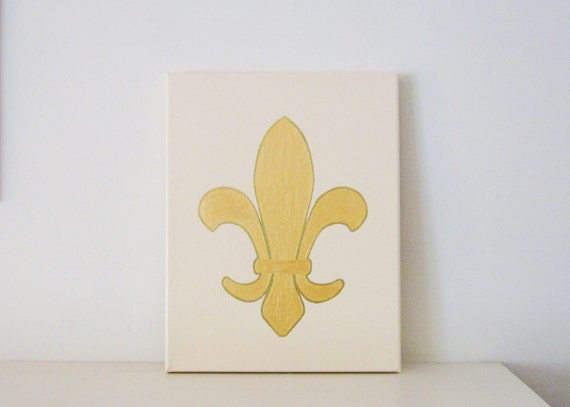This image is a color photograph capturing a rectangular canvas featuring a hand-painted gold fleur-de-lis, which resembles the hue of a ripe mango. The fleur-de-lis, a trifoil symbol with a central upright point flanked by two side points that curve outward and downward, is set against a beige background. The artwork is perched on a white table, and both the table and the canvas are placed against a white wall, adding to the simplicity of the scene. The brushstrokes of the painting hint at its handcrafted nature, evident by its slight asymmetry. Overall, the scene is minimalist, focusing primarily on the gold fleur-de-lis.